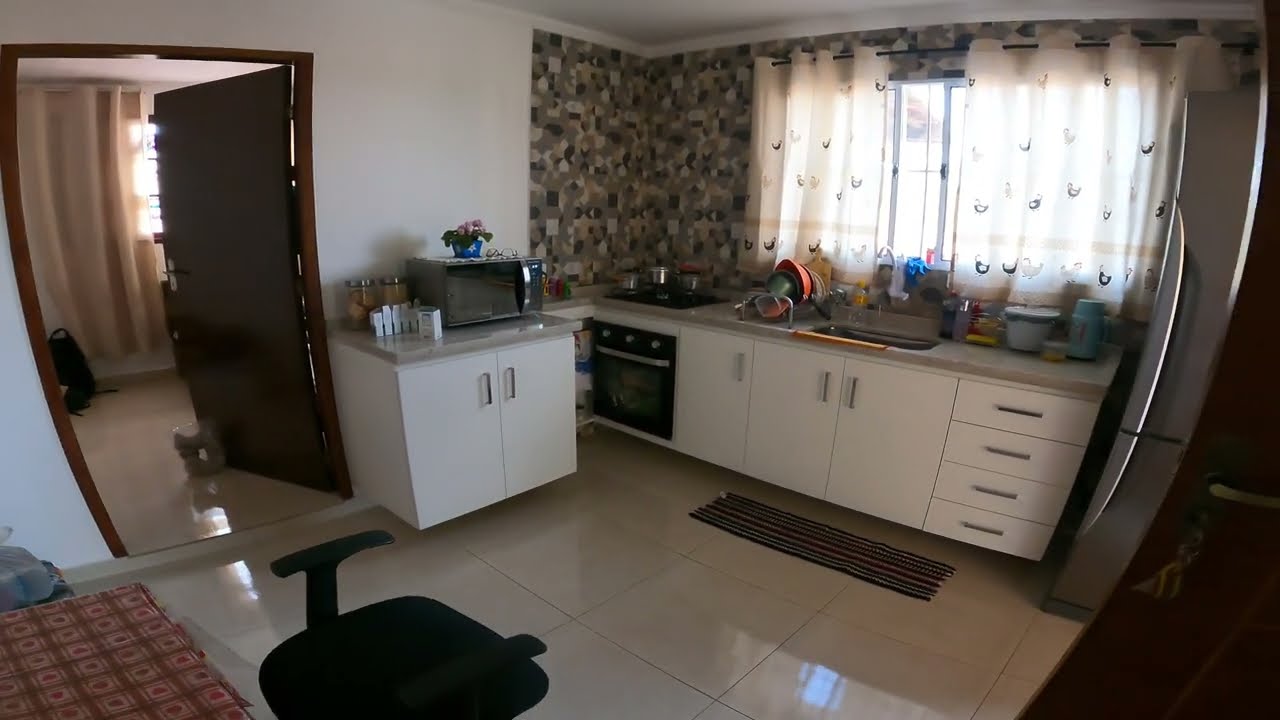The image captures an interior view of a kitchen marked by white cabinets with silver handles and tan countertops. A deep sink sits centrally, flanked by dishes drying on the left side, and a thin, striped rug lies on the floor in front. The backdrop features a stone-patterned backsplash in varied shades of white and gray, adding texture and contrast. To the right, a metallic-colored refrigerator stands prominently. The left side of the image reveals an open brown door leading into a bedroom, where a backpack rests against the wall and a tan-colored curtain hangs, partially covering the window. Additionally, a red-checkered tablecloth and a backless black computer chair can be seen near the doorway. The room's floor is made of large white tiles, and light filters faintly through the gauzy, closed curtains above the sink, contributing to the overall ambiance.